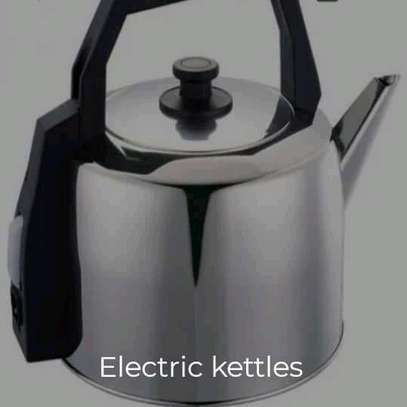The image features a sleek, stainless steel electric kettle with a reflective silver surface, set against a light grayish-blue background. The kettle has a rounded, almost marshmallow-like shape with a flat bottom. Prominently displayed in white text on the lower part of the kettle are the words "electric kettles." The spout, which is positioned on the right side, is smooth and extends vertically. The black handle, made of thick plastic, runs straight up, across, and back down, incorporating a black plastic section with a gray button for operational control. The top of the kettle features a black knob on the lid, allowing for easy removal. Notably, the sides of the kettle slightly reflect the surrounding light, adding subtle highlights to its polished surface.